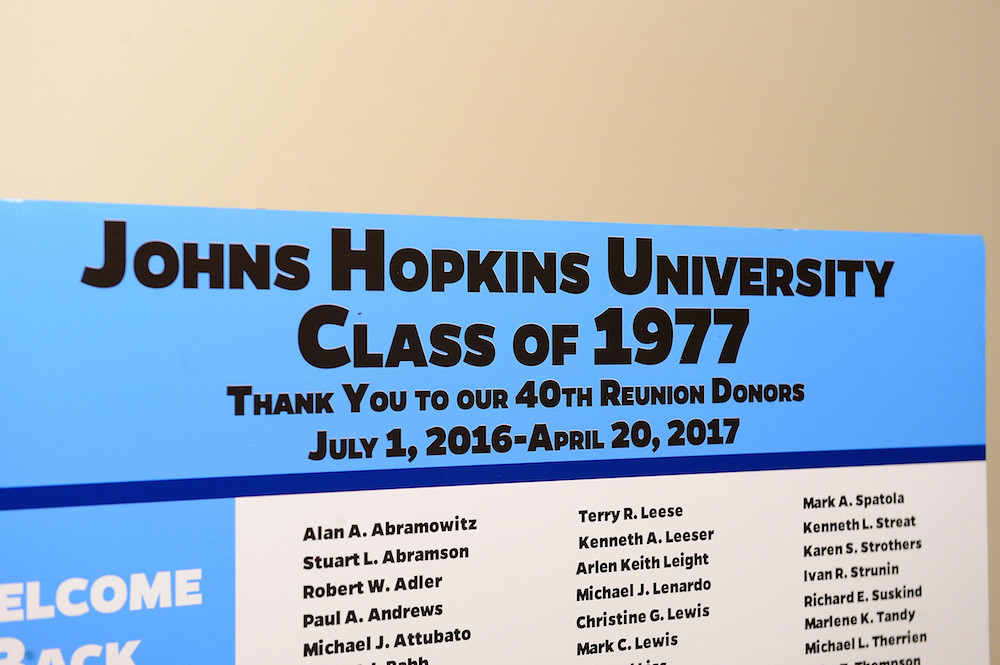The image showcases a vividly-colored sign in blue, light blue, black, and white hues, affixed to a wall under bright natural light. The top of the sign bears the heading "Johns Hopkins University Class of 1977" in bold font, followed by a message of gratitude: "Thank you to our 40th reunion donors July 1st, 2016 to April 20th, 2017." Beneath this message is a list of names of the generous donors, although the list is partially cut off at the bottom. The visible names include Alan A. Abramowitz, Stuart L. Abramson, Robert W. Adler, Paul A. Andrews, Michael J. Atubado, Terry R. Leis, Kenneth A. Leiser, Arlen Keith Leite, Michael J. Leonardo, Christine G. Lewis, Mark C. Lewis, Mark A. Spatola, Kenneth L. Street, Karen S. Struthers, Ivan R. Struden, Richard E. Suskind, Marlene K. Tandy, and Michael L. Sarian, arranged from left to right. The bottom left corner of the sign, partially obscured, appears to warmly greet alumni with the phrase "Welcome back." The clarity of the image enhances the visibility of all these details.